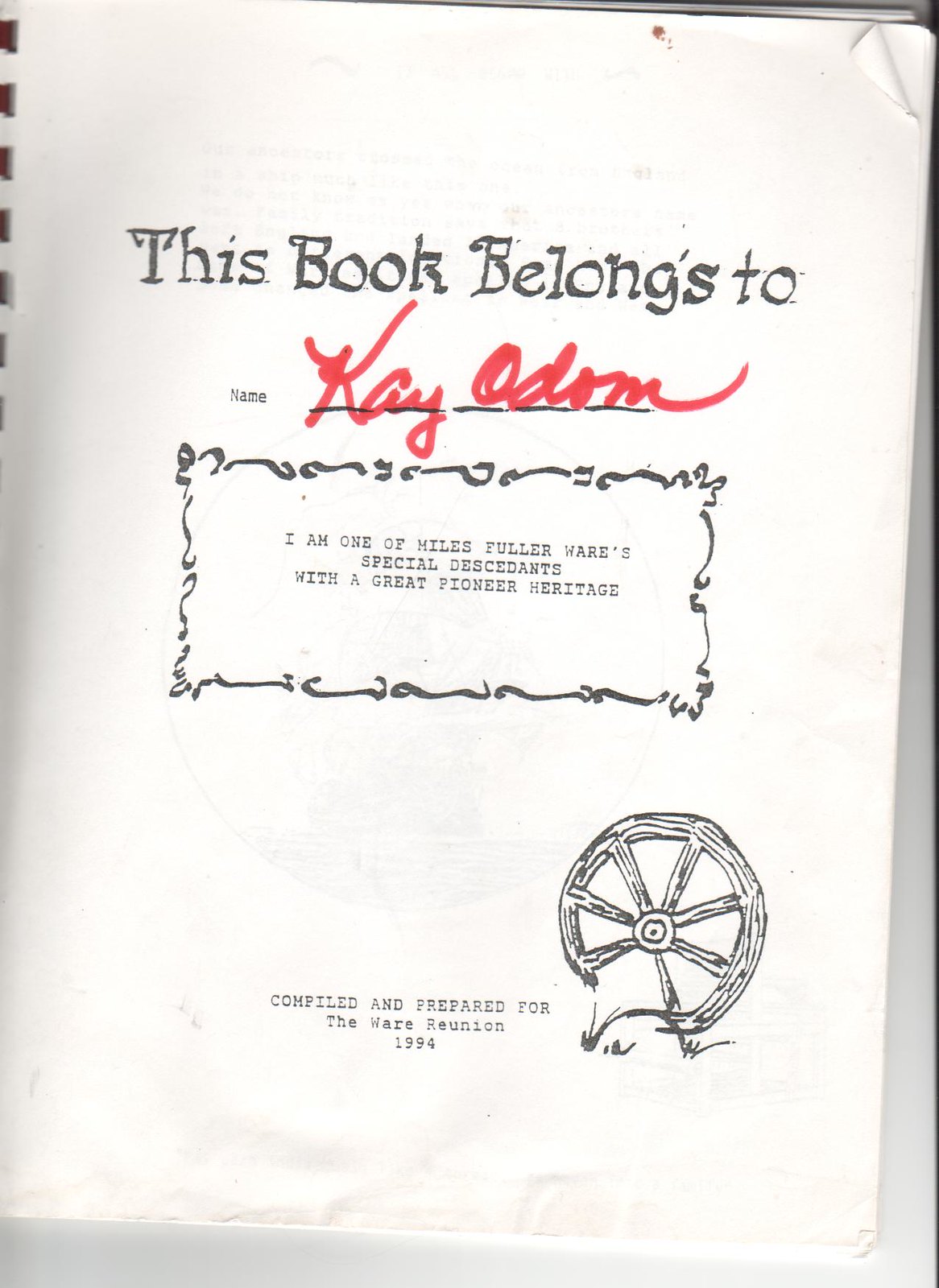The image depicts the cover page of a book prepared for a family reunion, likely produced at a copy shop and bound with a plastic spiral. The grainy cover, suggesting it might be a photocopy, features a headline at the top that states, "This book belongs to." Beneath this, in red cursive writing, is the name "K. Odom." Enclosed in a rectangular box with a squiggly line border, it declares in uppercase font, "I am one of Miles Fuller Ware's special descendants with a great pioneer heritage." In the lower right corner, there is a clip art drawing of a black and white wagon wheel, partly obscured by a rock. To the immediate left of the drawing, the text reads, "Compiled and prepared for the Ware Reunion, 1994." The entire cover page is rendered in black and white, except for the red ink used for the name "K. Odom," and showcases the era's typical design aesthetics.